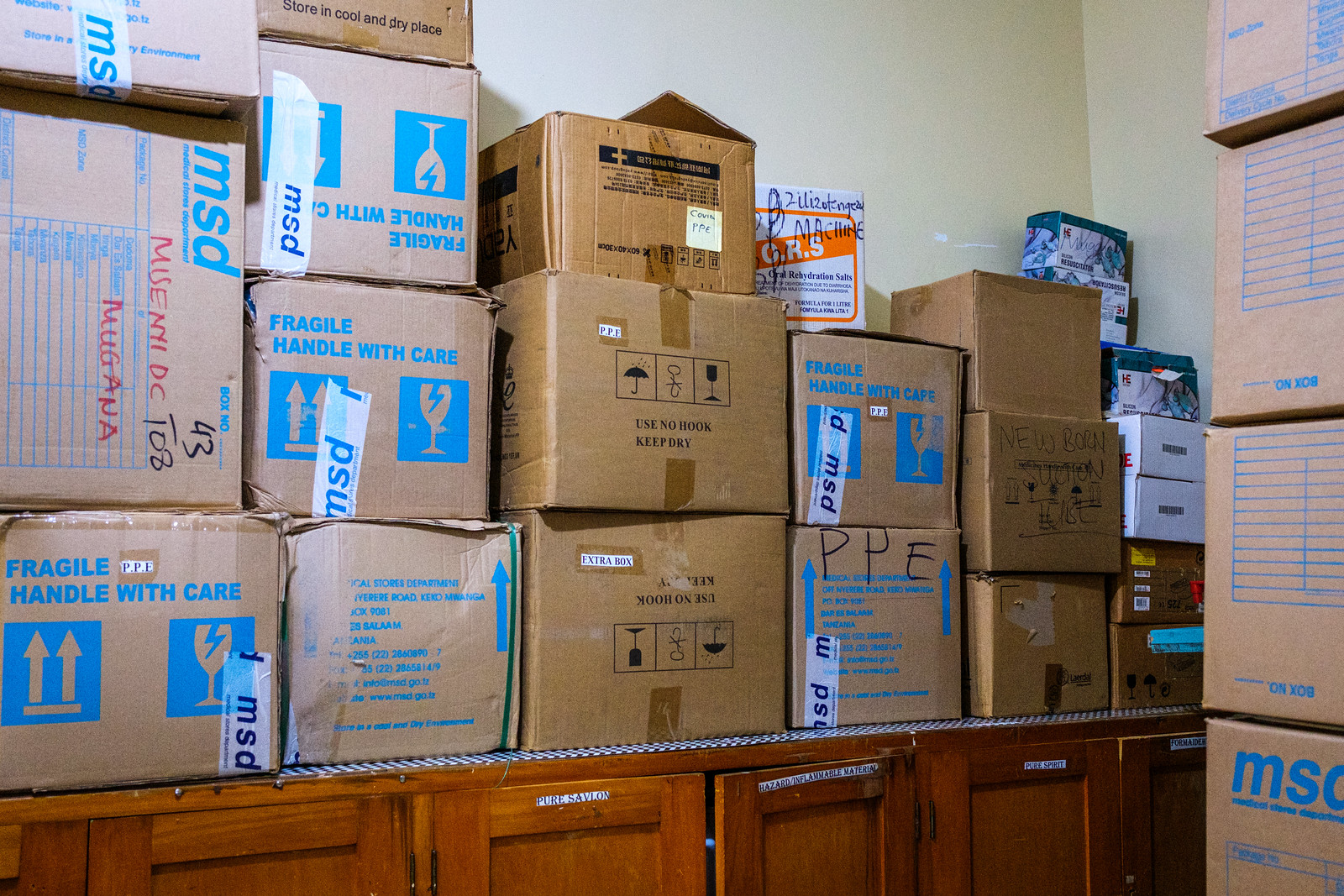The indoor image depicts a cluttered office or storage room featuring an assortment of objects and colors. At the bottom of the image, there is a brown, wooden cabinet with five visible doors. On the countertop above the cabinet are numerous cardboard boxes stacked haphazardly. These boxes vary in orientation, with some facing forward, some backward, and some on their sides. The boxes prominently display labels saying "Fragile, Handle with Care," and are marked with various blue and red symbols and text such as "MSD," "MUSNYDC," "MUGANA," and "PPE." Additionally, there are descriptions indicating medical items like "newborn suction tubes" and "oral rehydration salts." To the right side of the image, more cardboard boxes are stacked on the floor, with at least four larger boxes featuring blue lettering. The color palette of the image includes brown, light brown, blue, red, black, orange, teal, and yellow, with the beige walls forming the backdrop. Given the contents and setting, the space might be a hospital storage room. The scene conveys a sense of organized chaos typical of busy storage areas.